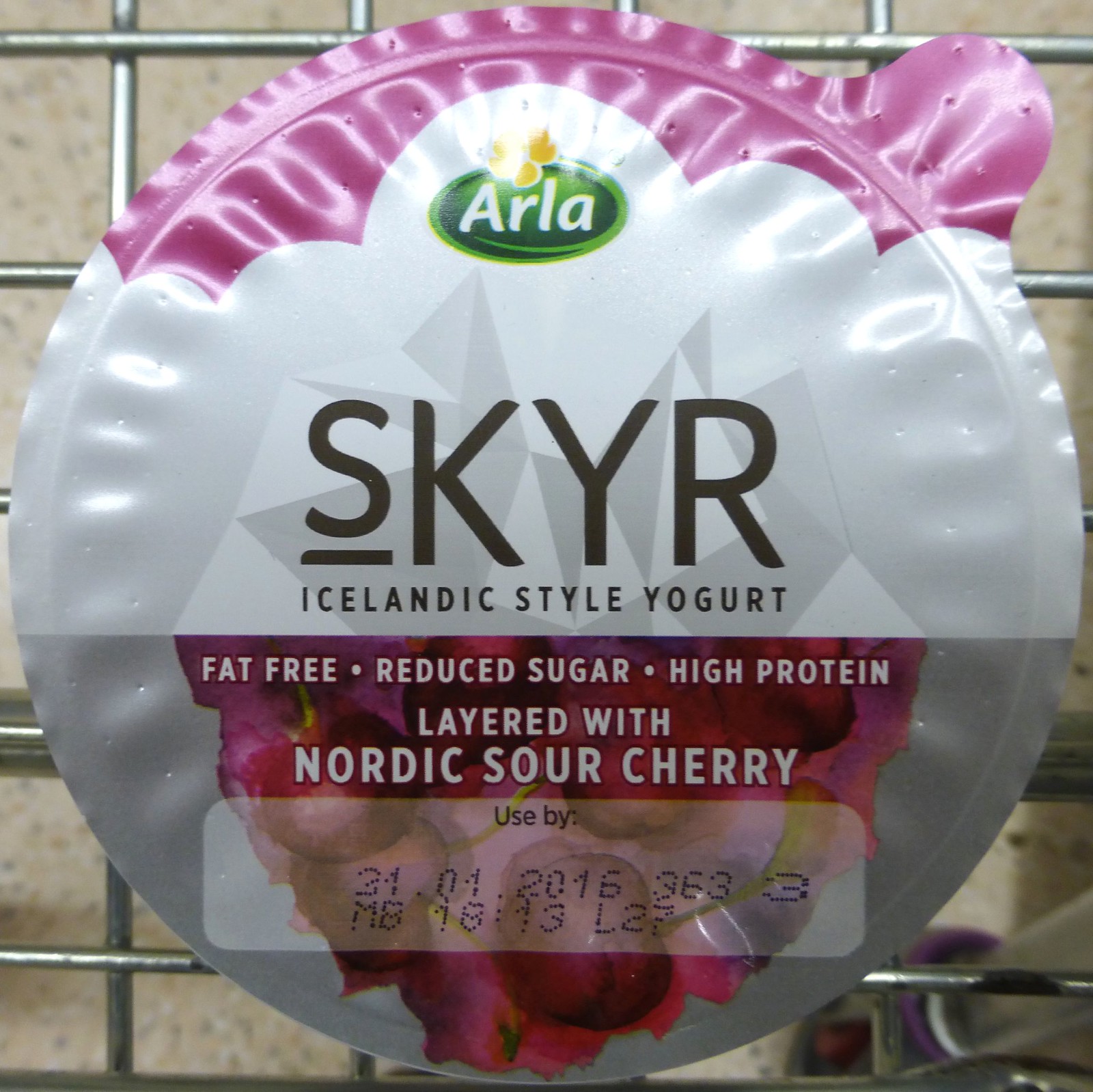This image shows a close-up of the lid of an Arla yogurt container. The lid features a white background with accents in purple and pink. Dominating the design is the Arla logo: the word "Arla" in white lettering set against a green background with a small yellow flower. Below the logo, bold letters spell out "SKYR," and in smaller, all-uppercase letters, it reads "ICELANDIC STYLE YOGURT." Further down, the text highlights key product features: "FAT-FREE," "REDUCED SUGAR," and "HIGH PROTEIN." Notably, the yogurt is described as "LAYERED WITH NORDIC SOUR CHERRY." At the bottom of the label, there's a use-by date, marked "USE BY 21.01.2016," along with the code "S633MB1813L27." The lid is shown leaning against a metal grid, with a beige wall visible in the background.